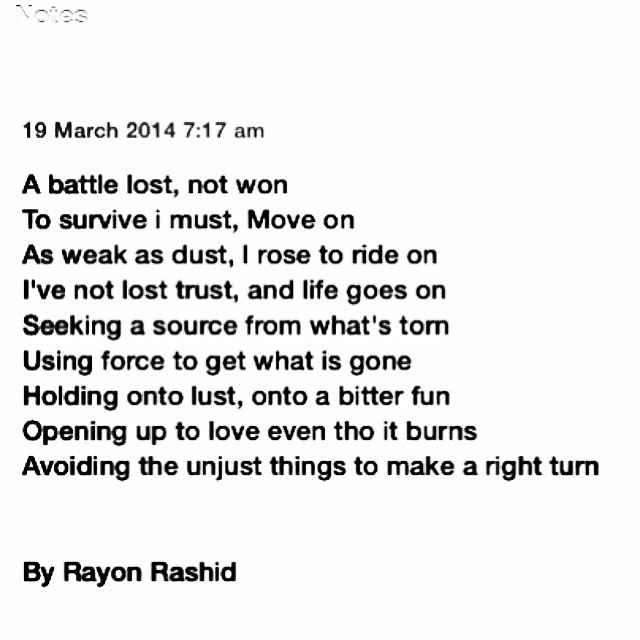This image captures a monochromatic screenshot, likely from a smartphone's notes application, showcasing a poem written by Rayon Rashid. The background is entirely white, while the text appears in black, creating a stark contrast. At the very top, the word "Notes" is faintly visible in gray, suggesting it was written on a notes app. Below the header, the date and time "19 March 2014, 7:17 AM" are prominently displayed. The poem, presented just beneath this timestamp, reads: 

"A battle lost, not won.  
To survive, I must move on.  
As weak as dust, I rose to ride on.  
I've not lost trust, and life goes on.  
Sourcing a source, seeking a source from what's torn.  
Using force to get what is done.  
Holding on to lust, onto a bitter fun.  
Opening up to love, even though it burns.  
Avoiding the unjust things to make a right turn."  

The author's name, Rayon Rashid, is inscribed at the bottom, further indicating its authorship. There are no additional images or graphics, leaving the powerful words of the poem as the sole focus of this minimalist yet poignant image.